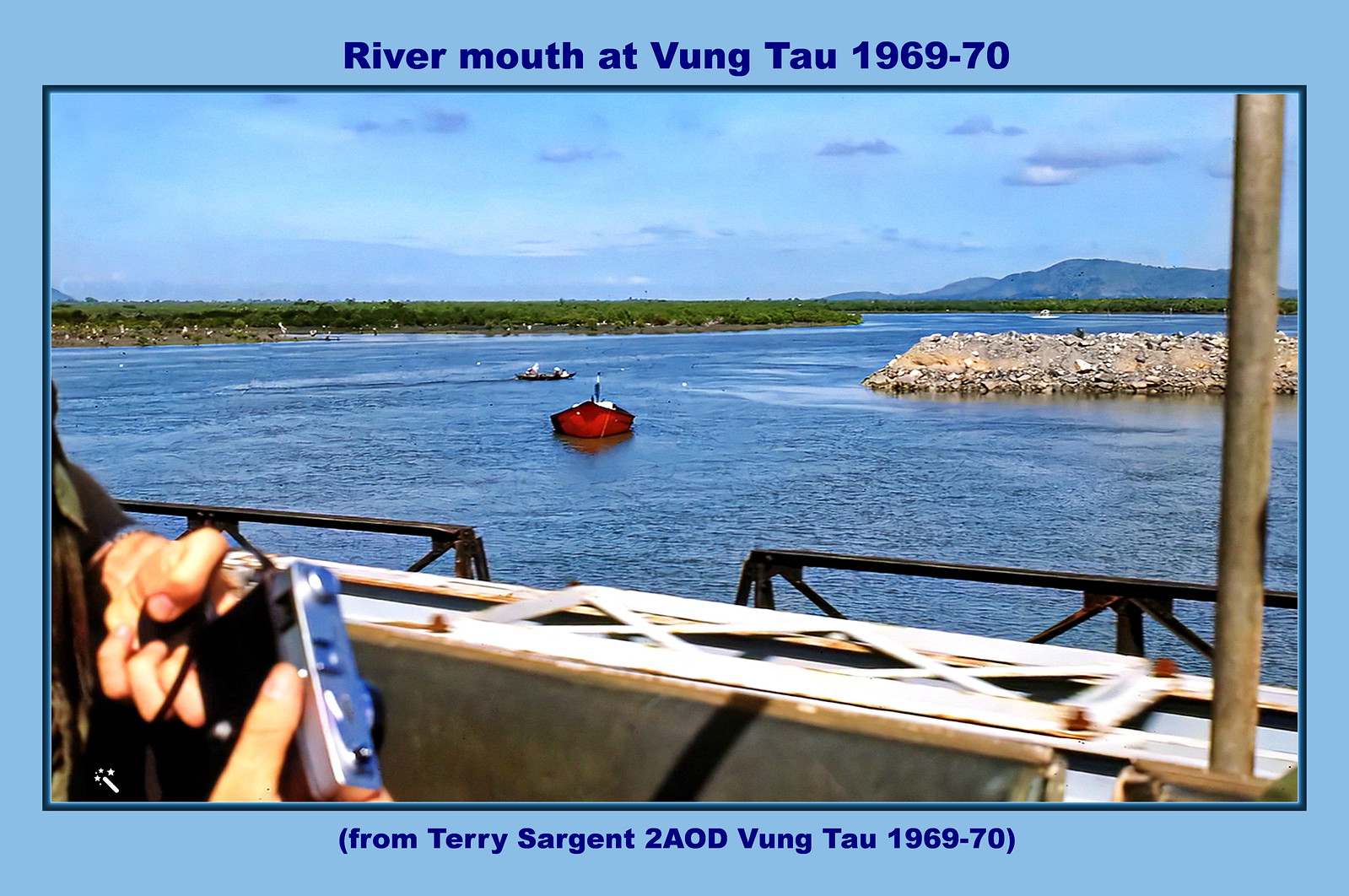The image features a historical photograph bordered by a light blue frame, inscribed with the text "Rivermouth at Vung Tau, 1969-70. From Terry Sargent to AOD, Vung Tau, 1969-70." At the center of the photograph is a river mouth scene in Vietnam dated from 1969 to 1970. The photograph shows a large river with one prominent boat fairly centered in the image, painted red, and accompanied by smaller, less discernible boats scattered in the background. The viewer's perspective seems to be from another boat or a platform, as evidenced by a person's hands holding an old camera at the bottom left corner. Distant shores are visible, adorned with green grass, and mountain ranges stretch across the horizon. The scene is illuminated by daylight, evoking a clear outdoor setting with hints of wildlife, possibly birds, and a small land mound to the immediate right of the frame. The image palette includes light blue, dark blue, white, grey, green, red, tan, silver, and brown, capturing the nostalgic essence of this historic moment.